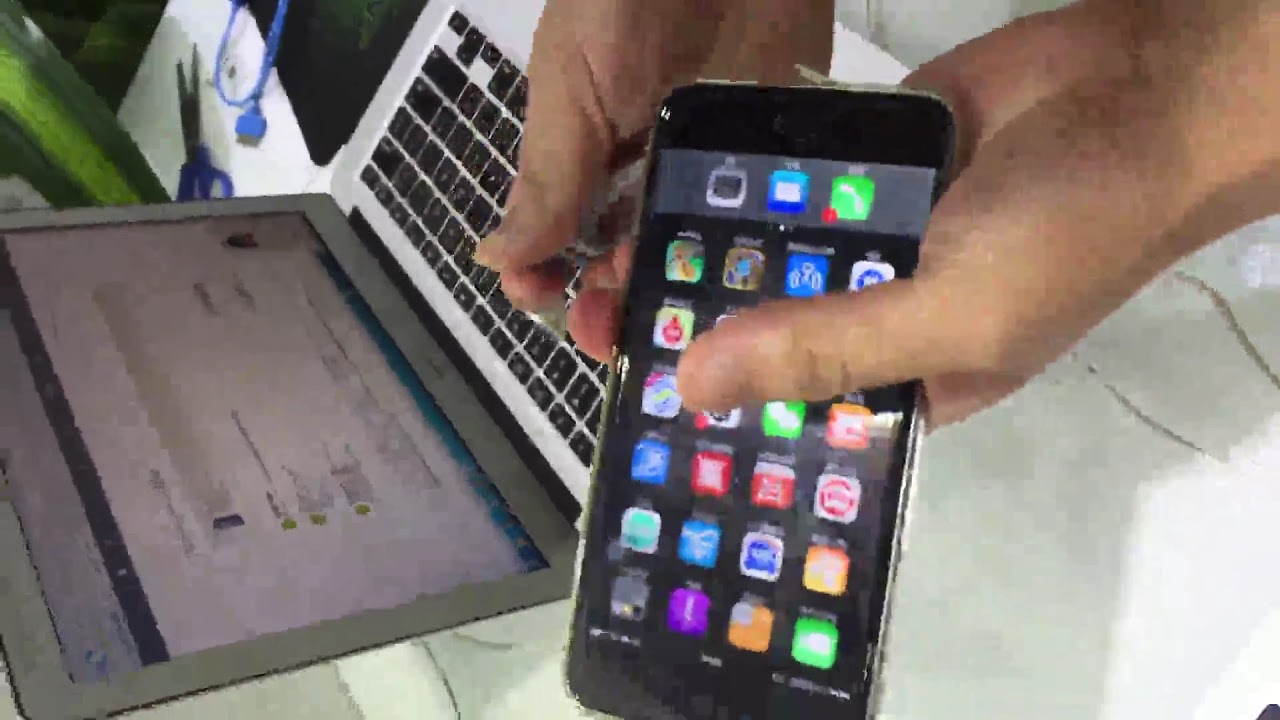In this indoor image taken on a white desk, light brown hands hold a large smartphone with a screen displaying colorful icons, possibly an iPhone. The phone is centered in the frame, casting a shadow from the top light source. To the left of the smartphone, a light gray or silver laptop with a silver keyboard and black keys is open, displaying an unreadable, blurry screen. Also on the desk are a pair of blue-handled scissors and a blue charging cable. The scene includes various colors, such as white, gray, green, orange, purple, blue, black, red, tan, and silver, hinting at a lively home office or workspace.